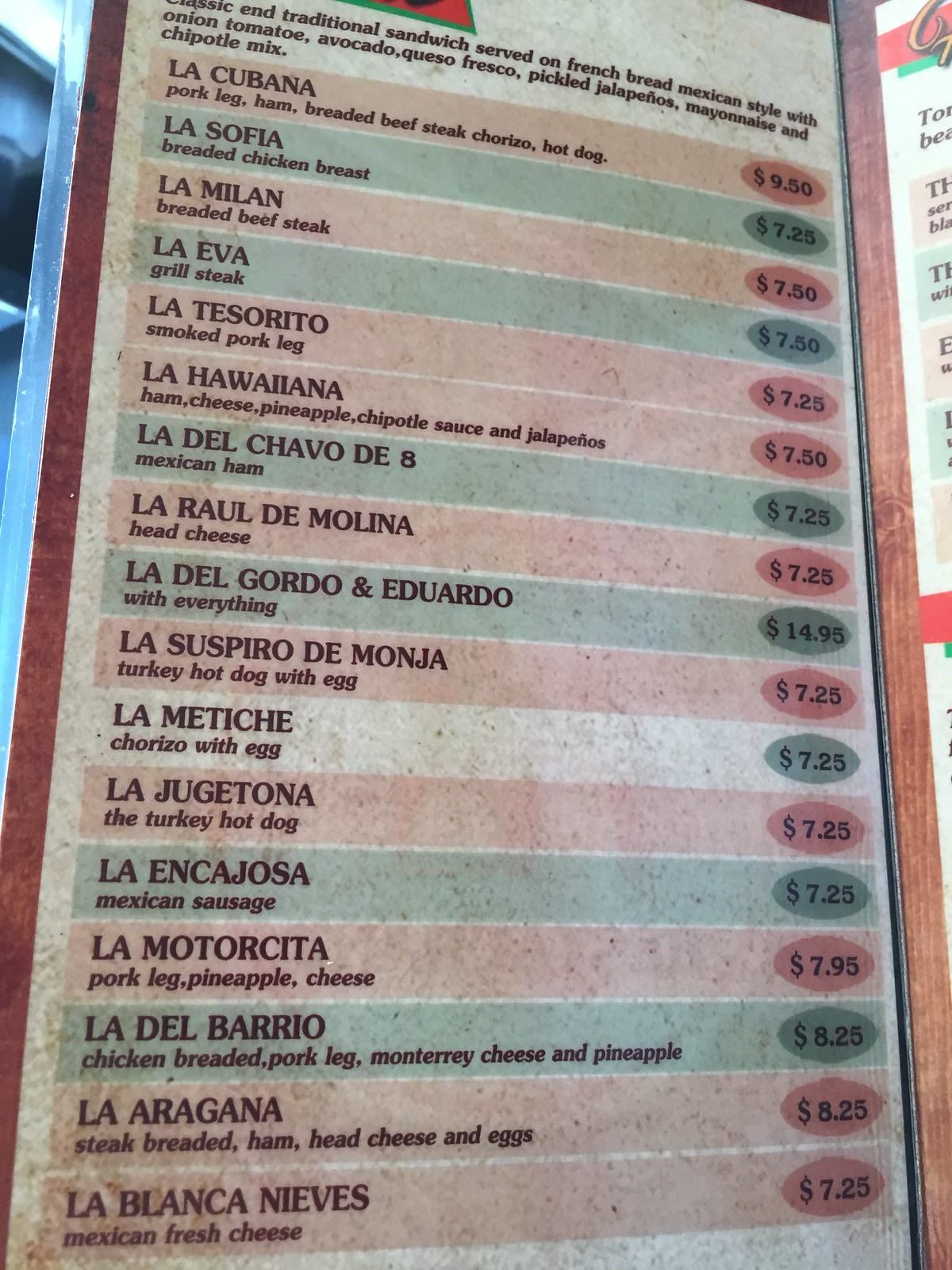Here is a detailed and cleaned-up caption for the given image description:

---

The image displays a vibrant menu set against a white background, adorned with alternating stripes predominantly in light pink and light green, with a single white stripe running down the middle. The text is in black font, predominantly in Spanish, listing an array of mouth-watering sandwich options. At the very top, black text on a white strip introduces the menu with the description: "Classic and traditional sandwiches served on French bread Mexican style with onion, avocado, queso fresco, pickled jalapeños, mayonnaise, and chipotle mix."

Highlighted in pink, the menu features the following sandwiches:

1. **La Cubana**: A hearty combination of pork leg, ham, breaded beef steak, chorizo, and hot dog for $9.50.
2. **La Sofia**
3. **La Milan**
4. **La Eva**
5. **La Tesorito**
6. **La Hawayana**
7. **La Del Chavo de Ocho**
8. **La Raul de Molina**
9. **La Del Gordo y Eduardo**
10. **La Suspiro de Monja**
11. **La Matiche**
12. **La Jugatona**

Each of these sandwiches likely offers unique and delicious ingredients, encapsulating various traditional and classic Mexican flavors.

---